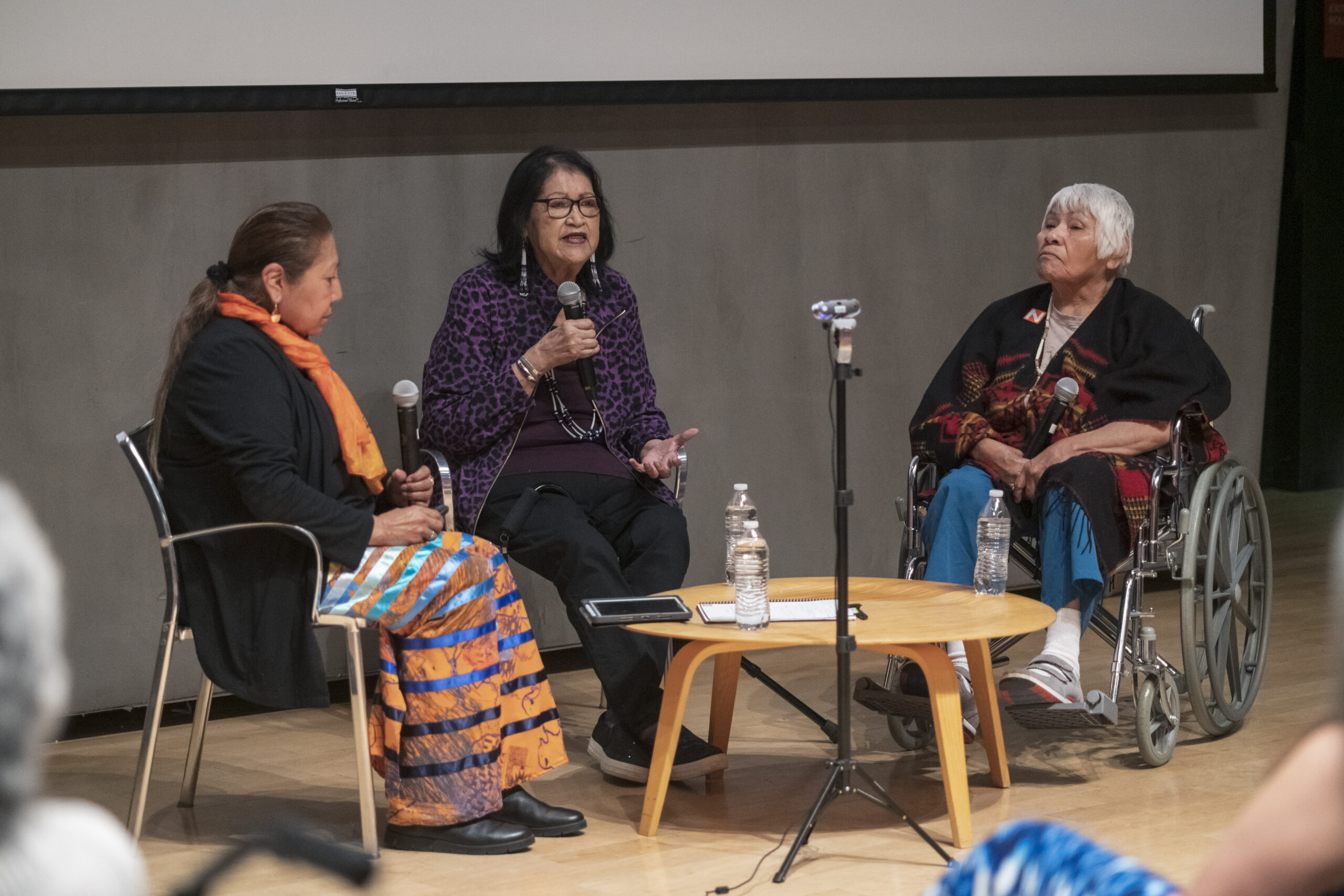The image captures three women sitting on a stage, each holding a microphone, likely participating in a conference or presentation. They are seated behind a small round wooden table that holds water bottles, a phone, and a clipboard. The woman on the far left has a long ponytail and brown hair, is dressed in a black jacket and orange dress with blue and metallic light blue stripes, complemented by black shoes, and wears an orange scarf. The middle woman, with short black hair, glasses, and long earrings, dons a purple and black animal print jacket, black pants, and black shoes. The woman on the far right, seated in a wheelchair, has very short white hair and looks proud. She is dressed in blue pants, a printed pullover, and shoes with red soles. Behind them, a projector sits unused, and the venue appears to be a theater or convention setting. The women may possibly be of Native American descent, though it's challenging to determine from the photo alone.